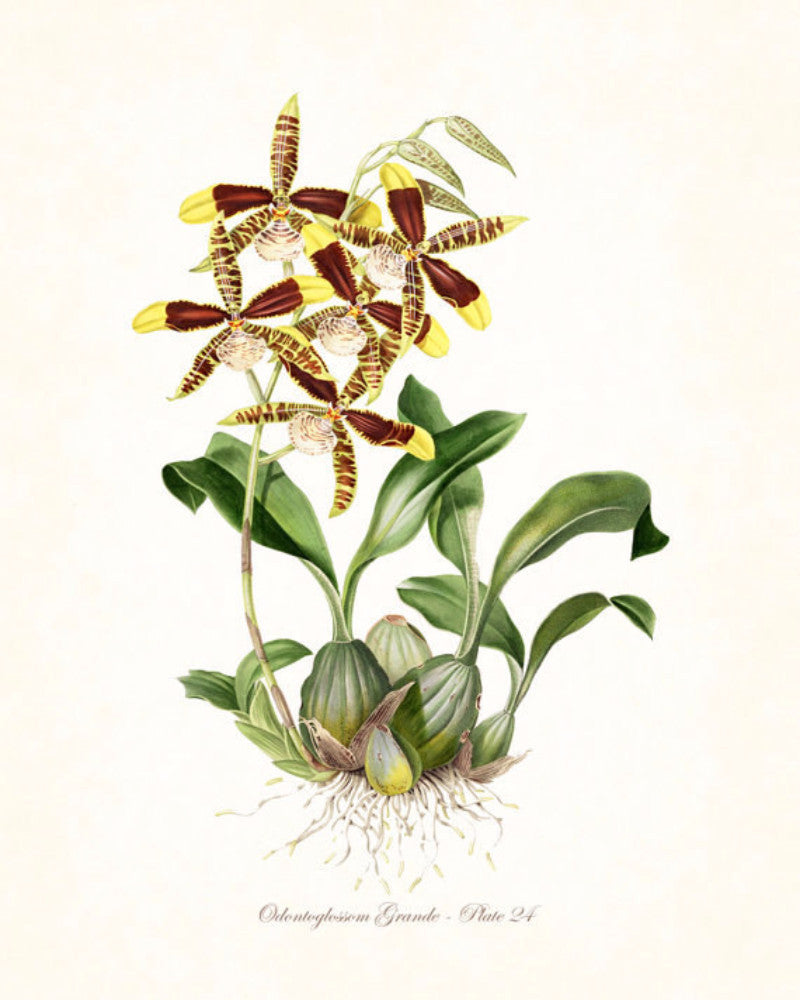The rectangular image, measuring approximately six inches high by four to five inches wide, features a delicate botanical illustration set against a very pale pink background. At the bottom center of the image, there is brown text reading "Odentic Trium Grande - plate 24." The striking focal point of the image is a detailed colored drawing of a plant, showcasing its entire structure from root to blossom.

The root system features thin, white, tentacle-like extensions tipped with yellow, anchoring the plant into the ground. Above the roots, there are three rounded green bulbous areas, each adorned with vertical striations. Two of these bulbous areas have sprouted long, slender leaves. To the left, a long green stalk with intermittent brown nodules rises from the ground.

Atop this stalk are unusual flowers with five elliptical petals. Two of the petals have a reddish-brown hue that transitions to golden yellow at the tips, while the other three exhibit a golden yellow base with horizontal reddish stripes. The flower's center features a fan-shaped bulb beginning with red stripes and fading to a clearish yellow hue.

The plant's enchanting, otherworldly appearance evokes a sense of curiosity and wonder, reminiscent of illustrations often found in science fiction narratives.